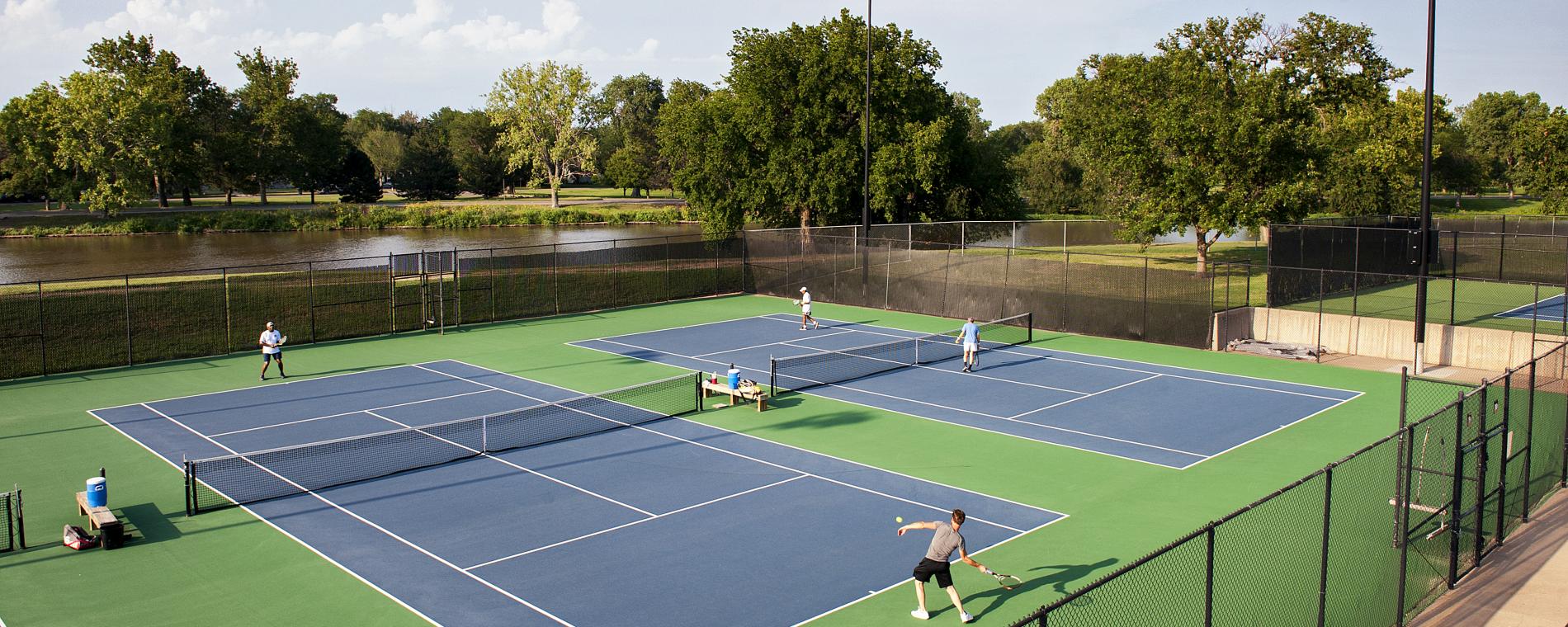The image is a detailed aerial view of two rectangular tennis courts in use, captured outdoors during the daytime. The courts, each painted in navy blue with white boundary lines, are surrounded by a tall black chain-link fence that forms a rectangular outline, extending from the bottom-right to the top-right and then across to the left-hand side of the image. Both tennis courts feature black nets spanning from the lower left to the upper right with players engaging in one-on-one matches on each court. The green ground encircles the courts with a vibrant grass-like appearance. Beyond the courts, a brown water body, likely a river or lake, stretches horizontally from left to right, bordered by a lush green field. The background is adorned with tall, dense trees under a partly cloudy blue sky, enhancing the photograph's scenic beauty.